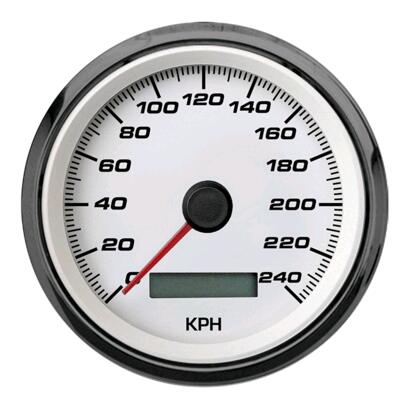This image features a close-up of a car's speedometer, isolated from the dashboard. The speedometer has a clean white background with black numerals and dash marks indicating speed increments. At the bottom, "kph" is clearly marked, denoting kilometers per hour. A small, non-backlit digital screen, intended to display the car's odometer reading, remains blank. The speedometer needle is currently positioned just below zero, giving the impression of a negative value. The numerals are styled in a sporty, square boxy font reminiscent of race car aesthetics. Encasing the speedometer is a dark silver bezel with varied reflective qualities, adding a subtle depth and shine.